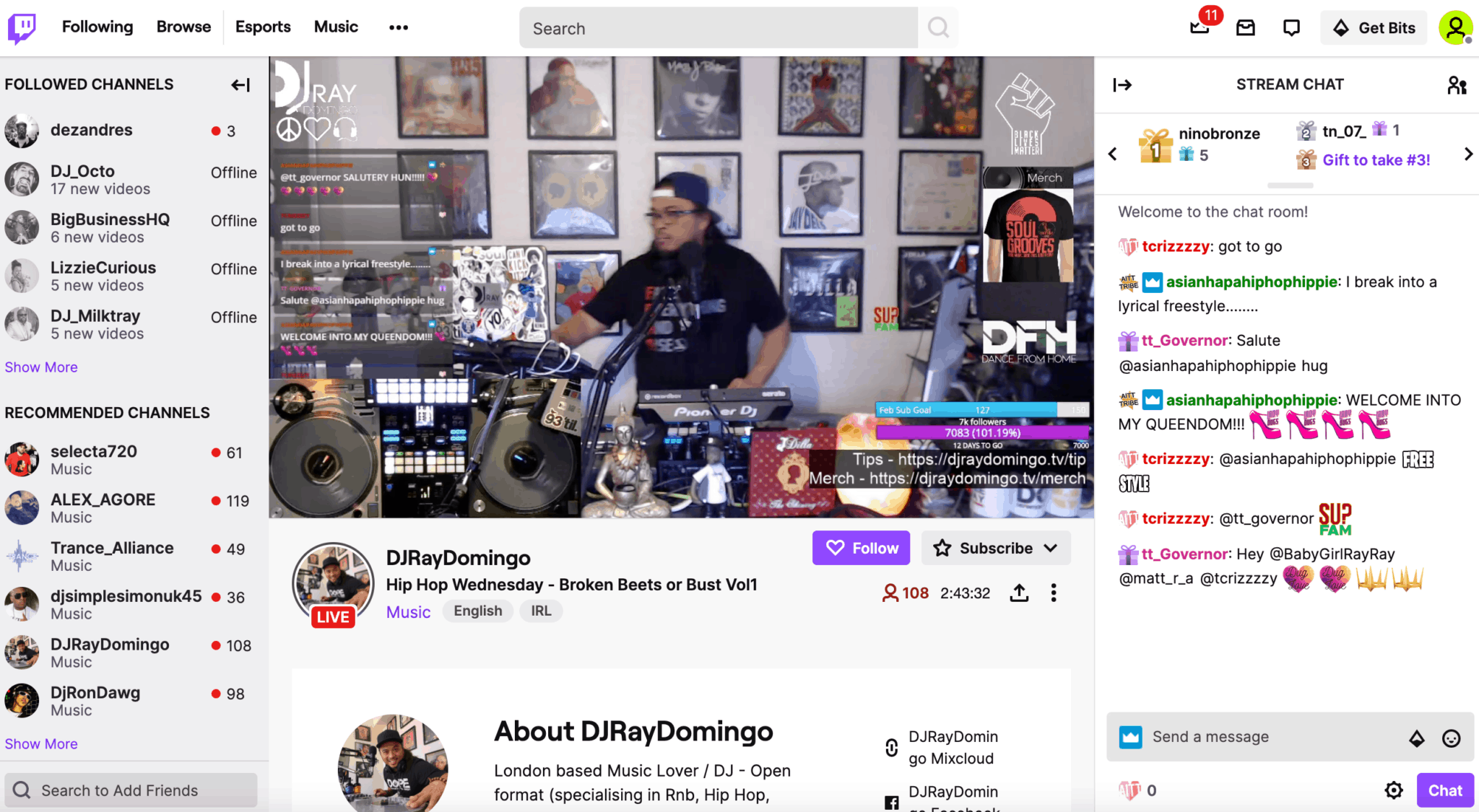This is a descriptive caption for a snapshot of a live Twitch stream:

At the top left of the screen, the iconic Twitch logo is prominently displayed. The central portion of the screen is occupied by a live video feed of a 25-30 year old man, appearing to be of Hispanic or Indian descent, with darker skin. He is in a cramped and crowded room, actively DJing using a combination of software and hardware, including turntables. Behind him, a white wall is adorned with framed album posters featuring iconic rap and R&B albums from the '90s, such as Nas's "Illmatic," A Tribe Called Quest's "Midnight Marauders," and Wu-Tang Clan's "Enter the Wu-Tang (36 Chambers)," among others.

On the far left, the Twitch interface displays an option to follow channels, listing five channels: Dr. Octo, Big Business HQ, Lizzy Curious, and DJ Milk Tray. Below this section, a list of recommended channels appears, including Selecta 720, Alex Agor, Trance Alliance, DJ Ray Domingo, and DJ Rondog, among others.

The stream image is identified as belonging to "DJ Ray Domingo," with the tag line "Hip Hop Wednesday, Broken Beats or Bust Volume 1" directly beneath his name. An "About" section follows, describing him as "London-based music lover, DJ, Open Format, specializing in R&B and Hip Hop."

On the far right side of the screen, the live stream chat is visible, buzzing with activity. At the top, it welcomes users to the chat room. The first visible message is from a user stating, "got to go," followed by another user named Asian Hip Hop Hippie, who says, "I break into a lyrical freestyle." The chat continues with various users exchanging greetings and quotes, contributing to the dynamic and interactive nature of the live stream.